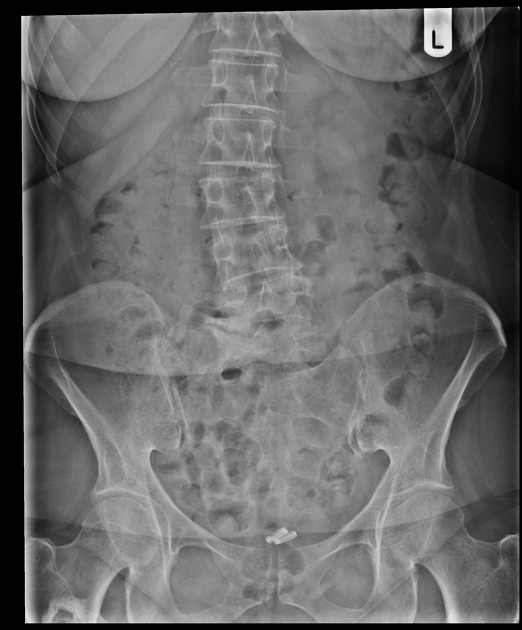This image depicts a vertically oriented, black-and-white x-ray of a person's torso. The x-ray is framed by a thin black border, which is most prominent on the left and top edges, while nearly non-existent on the right. A small white tag with a black capital letter "L" is visible in the upper right corner. Central to the image is the spine, with visible intervertebral discs, extending downward from the ribcage, which is faintly visible in the upper section, to the upper portion of the pelvis. The x-ray captures the lower chest, abdomen, and hips, revealing the curved outlines indicative of the lower breasts at the top of the image. Notably, near the bottom center, within the pelvic region, there are two distinct, pill-shaped white objects, possibly capsules, located where the uterus or bladder might be situated.